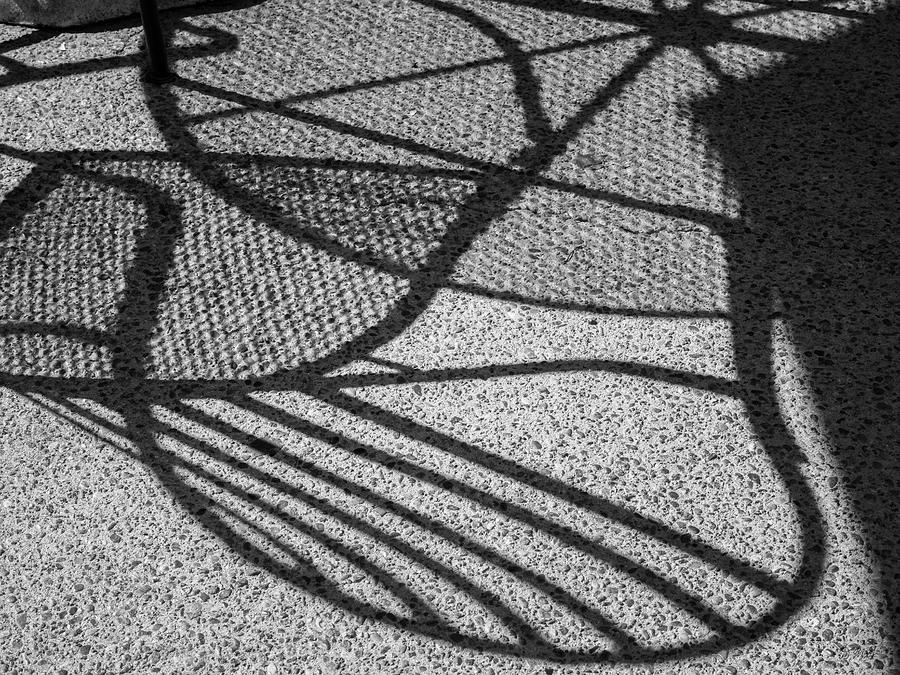This black-and-white photograph showcases the textured concrete floor of an outdoor patio. The concrete, embedded with various dark stones, has a smoothed, scrabble-like finish that is visually striking in its light gray tone. Shadows from the patio furniture create an intricate play of light and dark on the ground. At the top, a round table casts a shadow that is only partially visible, with its thin, wheel-like design evident. In the middle, the shadow of a patio chair is highlighted, featuring vertical slats that resemble a ladder or steps, and a mesh seat adding a complex texture to the shadow's pattern. To the right, a large, obscured rectangular shadow adds depth, contributing to the overall artistry of the scene. The light source from above casts these shadows crisply, emphasizing the detailed interplay between the furniture and the pebbled concrete below.